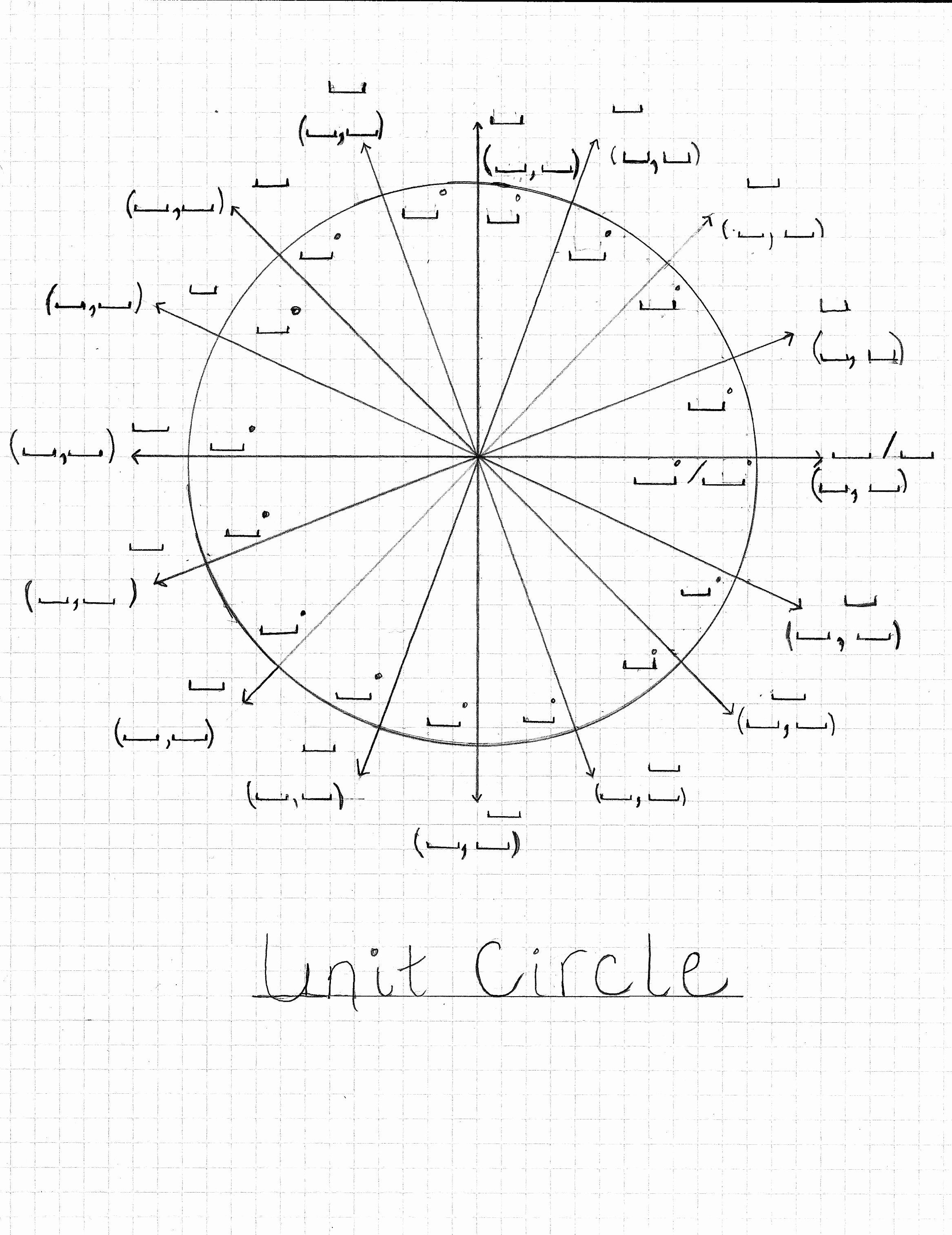The image is a black and white sketch of a unit circle, as labeled at the bottom in handwritten text, which is underlined. The background resembles a faded piece of grid paper, like you would use in math class, with faint black lines. At the center of the page is a large circle with numerous lines, specifically 16, radiating outward from a central point, resembling a pie chart. These lines turn into arrows that extend beyond the circle and point to illegible scribbled words. The arrows are equidistant from one another, creating an evenly spaced, symmetrical pattern.